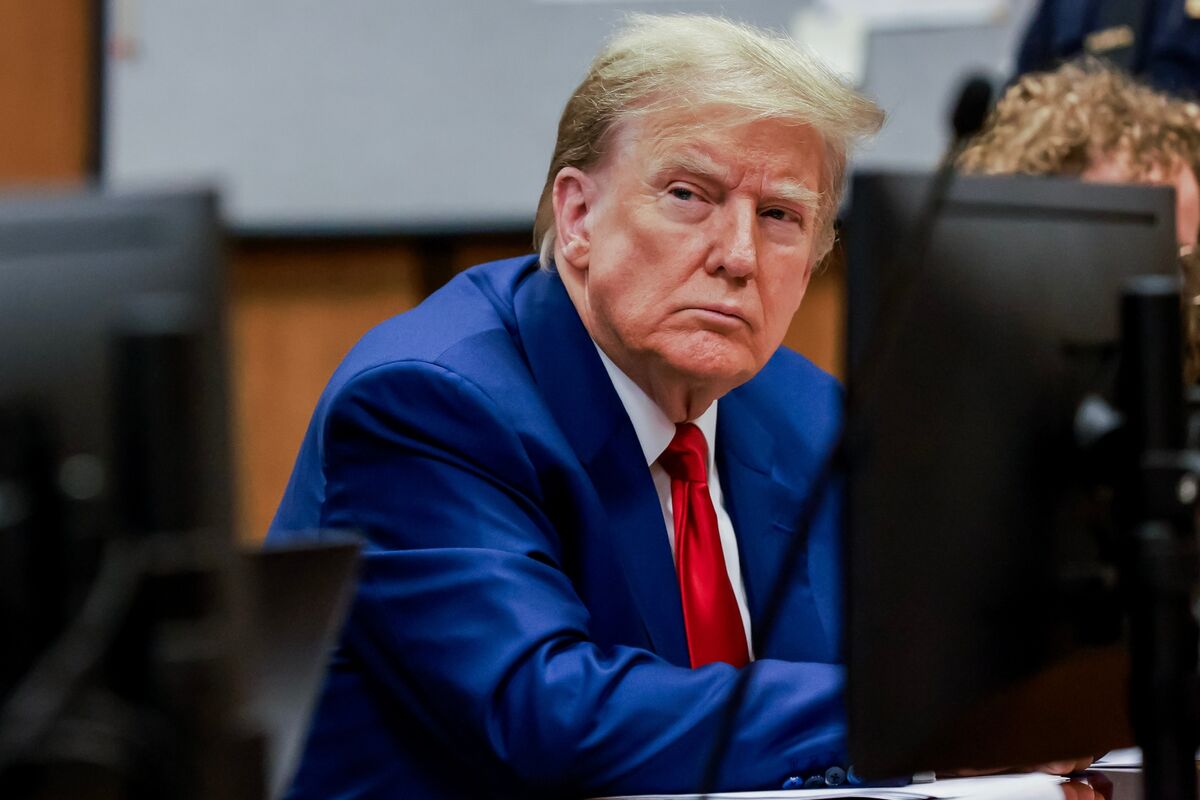The image features Donald Trump, likely in a courtroom setting, dressed in a bright blue suit, a white shirt, and his signature red tie. Trump, with his distinctive blonde hair, appears grumpy and is looking off to the side, possibly deep in thought. In front of him are black computer monitors, and behind him, a whiteboard with a black frame and some wood paneling. Next to Trump, on his left, is a person with curly brown hair and possibly glasses, only partially visible from the forehead. The colors in the photograph include vivid blues, reds, whites, blondes, and various earthy tones like tans and browns. The image seems suitable for use on news sites or social media due to its clear depiction of Trump in a formal and possibly legal environment.